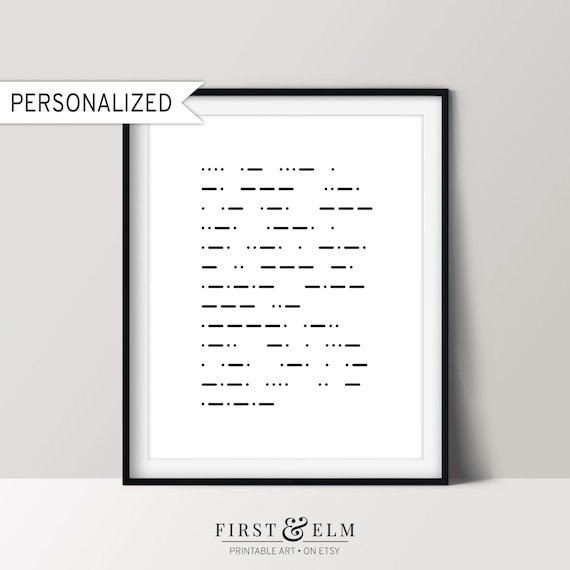This advertisement showcases a piece of framed art available on Etsy from a seller named First and Elm. The artwork features an off-white background with raised dashes and dots, resembling either Braille or Morse code, arranged in a text-like format. The image is enclosed in a thin black metal frame with a white photo matting. A banner across the top of the frame reads "personalized" in black letters on a white background, indicating that this artwork can be customized. At the bottom of the frame, the text "First and Elm, printable art on Etsy" is displayed in black letters. The entire ad is set against a gray background.